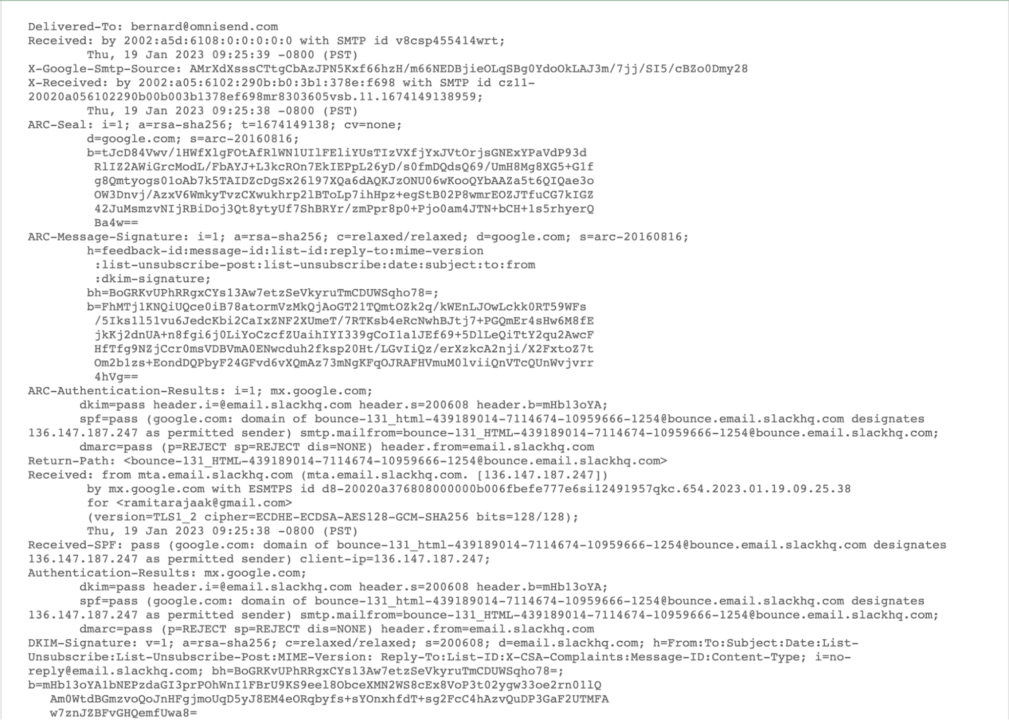This screenshot captures a detailed log of an email's journey through various servers, signifying a focus on network security or IT-related processes. The text is dense with technical jargon and alphanumeric sequences. Notable elements include:
- Delivery information: "Delivered to: Bernard at OmniSend.com"
- Receipt details: "Received by 2002:A5B:6108:: with SMTP ID"
- Security headers: "X-Google SMTP source," "ARC-seal," "ARC-message-signature," and "ARC-authentication-results"
- Multiple IP addresses are listed throughout the text.
- Other headers such as "Return-path," "Received," "Received-SPF," "DKIM-signature," and "List-Unsubscribe" are also visible.
This intricate log exemplifies the complex route and security checks an email undergoes before reaching its destination, underscoring the importance of these processes in maintaining cybersecurity integrity.